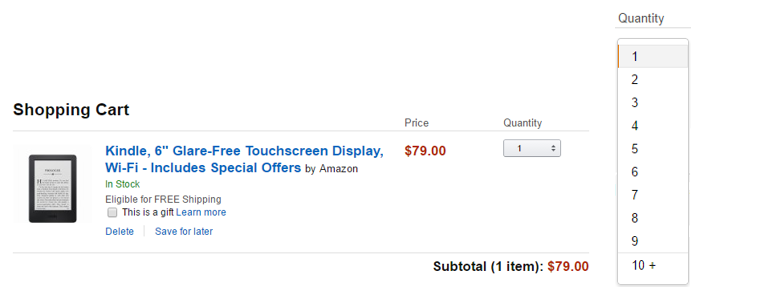This image is a screenshot of an Amazon shopping cart interface. The backdrop is clean and white, featuring the words "Shopping Cart" prominently on the left side. Below this header is a structured list of items currently in the cart.

Each item in the cart is presented with several key details:
- A small thumbnail image of the product.
- The product name.
- The manufacturer or brand name.
- Stock availability and shipping status.
- An option to mark the item as a gift.
- Links to delete the item or save it for later.

To the right of these details are the columns for the item's price and quantity. The quantity column features a dropdown menu, which in this screenshot is open, displaying options ranging from 1 to "10+". The current selection shows the quantity set to "1". 

At the bottom, beneath all listed items, appears the subtotal for the items in the cart, summarizing the total cost so far.